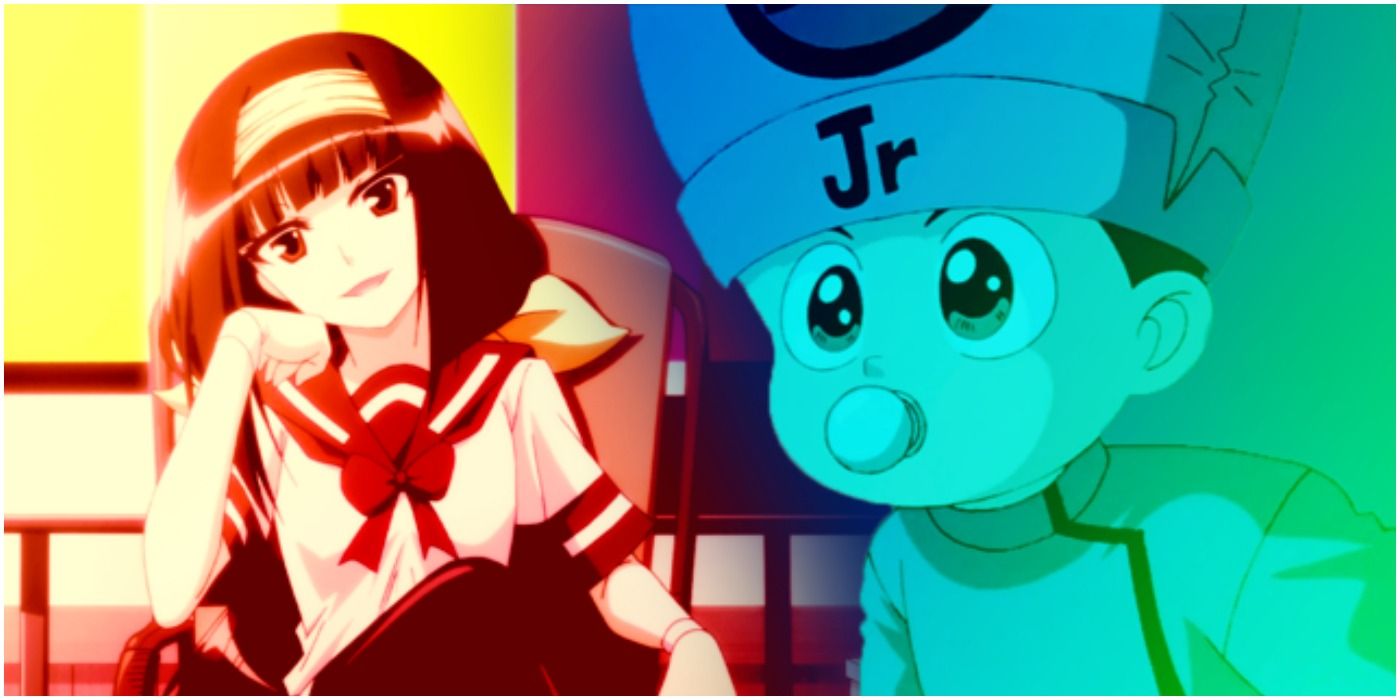This image is a detailed cartoon in an anime style, featuring two characters set against a colorful background. On the left, there's a young girl with long brown hair tied back with a yellow headband. She wears a sailor outfit with a white blouse accented by a red collar, a red necktie, and red stripes on her short sleeves. The girl is seated in a brown wooden chair, propping her hand under her chin, and she gazes with a hint of annoyance at the other character. Her expression is framed by a yellow backdrop that complements her silhouette.

On the right side of the image, there is a caricature of a little boy with exceptionally large eyes and a small, bulb-like nose. He wears a blue hat emblazoned with the black initials "JR," potentially signifying "Junior." The boy appears to be blowing a bubble, indicated by his pinky finger in his mouth. His attire consists of a green shirt with a white stripe, and the background behind him transitions from light green to blue, with indistinct reddish elements, possibly suggesting objects or abstract shapes. The overall scene juxtaposes the girl's red and orange hues with the boy's green and blue tones, creating a vibrant and engaging visual narrative.